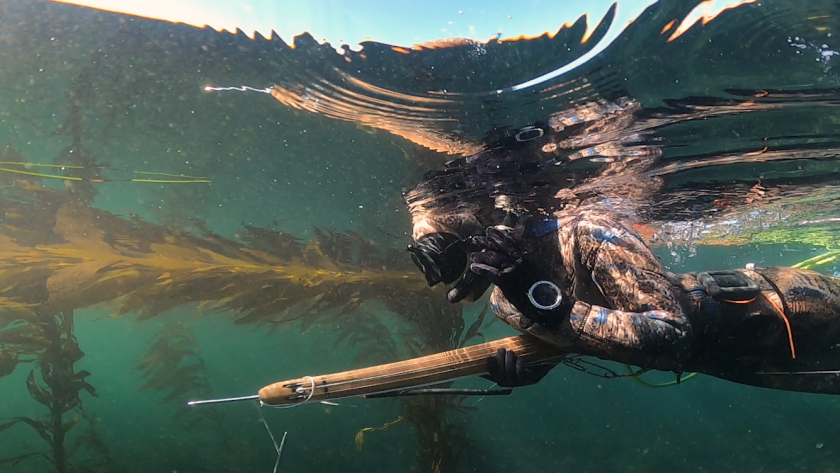In this underwater image, a woman is captured mid-dive, viewed from a side angle. She wears black goggles and has a black snorkel in her mouth, with the snorkel protruding to the water's surface. Her attire includes what appears to be a black wetsuit with mixed-pattern sleeves in gray, tan, and white hues. She also dons black gloves, with one hand holding the snorkel and the other gripping a wooden spearfishing gun, equipped with a long, sharp spear. The water around her has a greenish tint, and the background is filled with dark green and yellow-brown algae and seaweed. Above the water, the surface reveals a clear, light blue sky with sunlight glistening and creating ripples from her movements. The scene suggests she is either hunting or exploring in a vibrant aquatic environment.